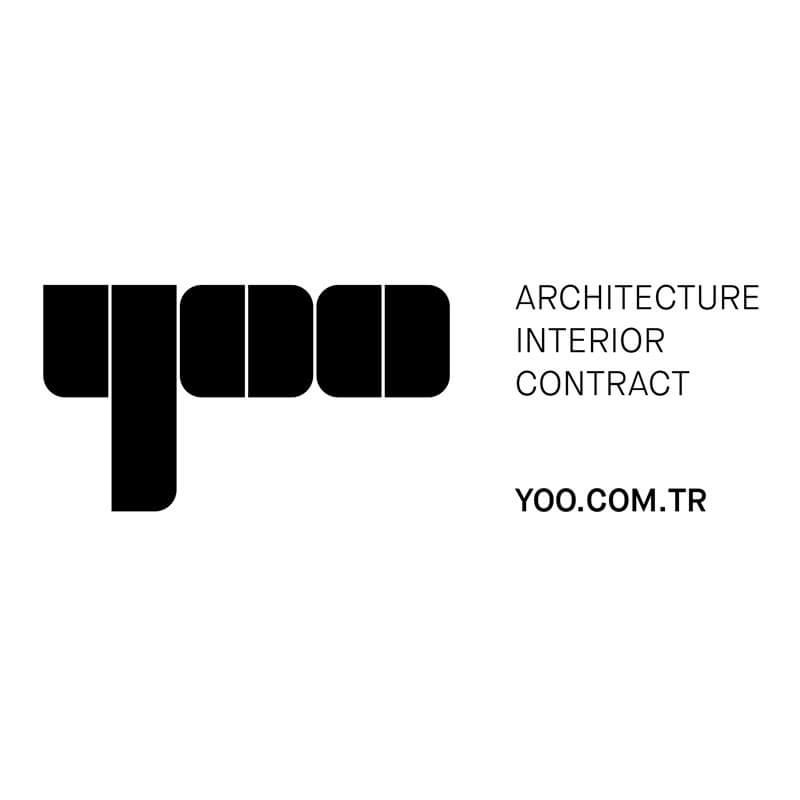The image features a logo set against a solid white background. On the left side, a bold, stylized black graphic forms the letters "YOO," representing the company's name. The design cleverly uses geometric shapes: one straight black stripe paired with a longer stripe creating a "Y," followed by mirrored curved stripes that form the double "O"s. To the right of this logo, three words—"ARCHITECTURE," "INTERIOR," and "CONTRACT"—are stacked vertically in thin black all-caps text. Below these words, in a more bold yet still smaller text, is the company’s website: "YOO.COM.TR." The overall composition is minimalistic and monochromatic, emphasizing the company's branding through simple yet striking design elements.